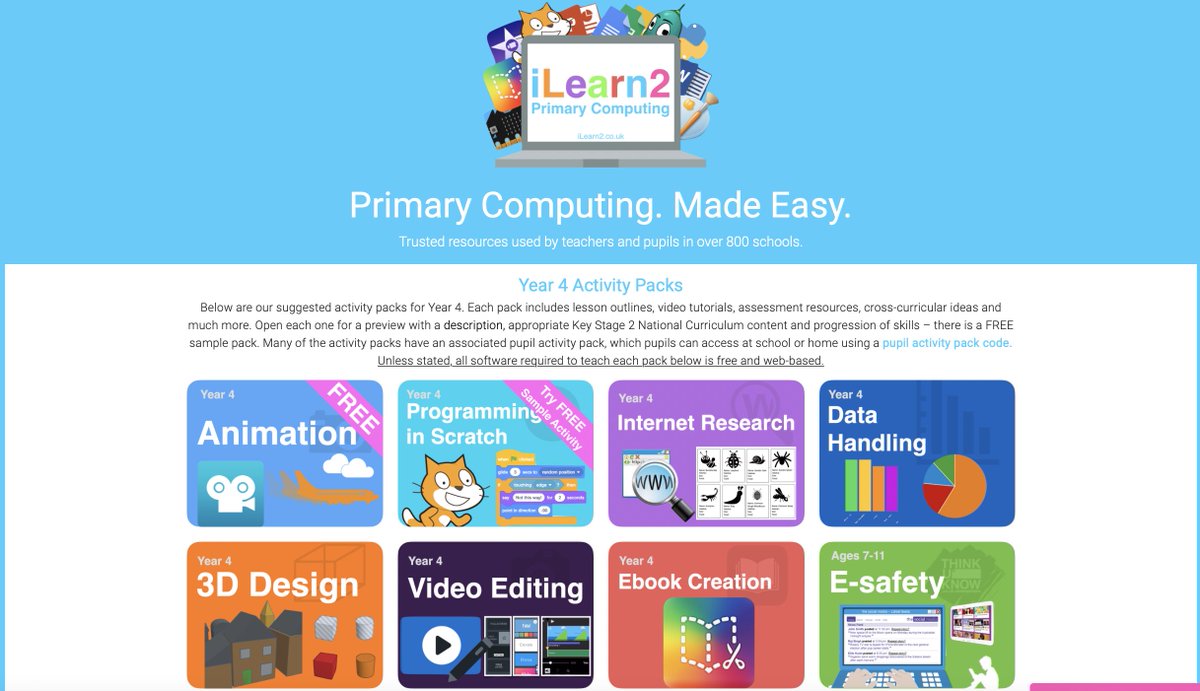At the top of the image, there is a wide blue bar featuring cartoon-style illustrations of books, tablets, and other kindergarten-related items. Within this bar, a monitor displays the text "iLearn2" (with a lowercase "i" and the digit "2"). Below the monitor, the text reads "Primary Computing." The main headline in large font states: "Primary Computing Made Easy: Trusted Resources Used by Teachers and Pupils in Over 800 Schools, Year 4 Activity Packs."

The image is further subdivided into sections highlighting the contents of the activity packs. There are four animated blocks in a single line, each representing a different component:
1. Animation
2. Programming and Scratch
3. Internet Research
4. Data Handling

Below this line, another set of four blocks showcases additional components:
1. 3D Design
2. Video Editing
3. eBook Creation
4. eSafety